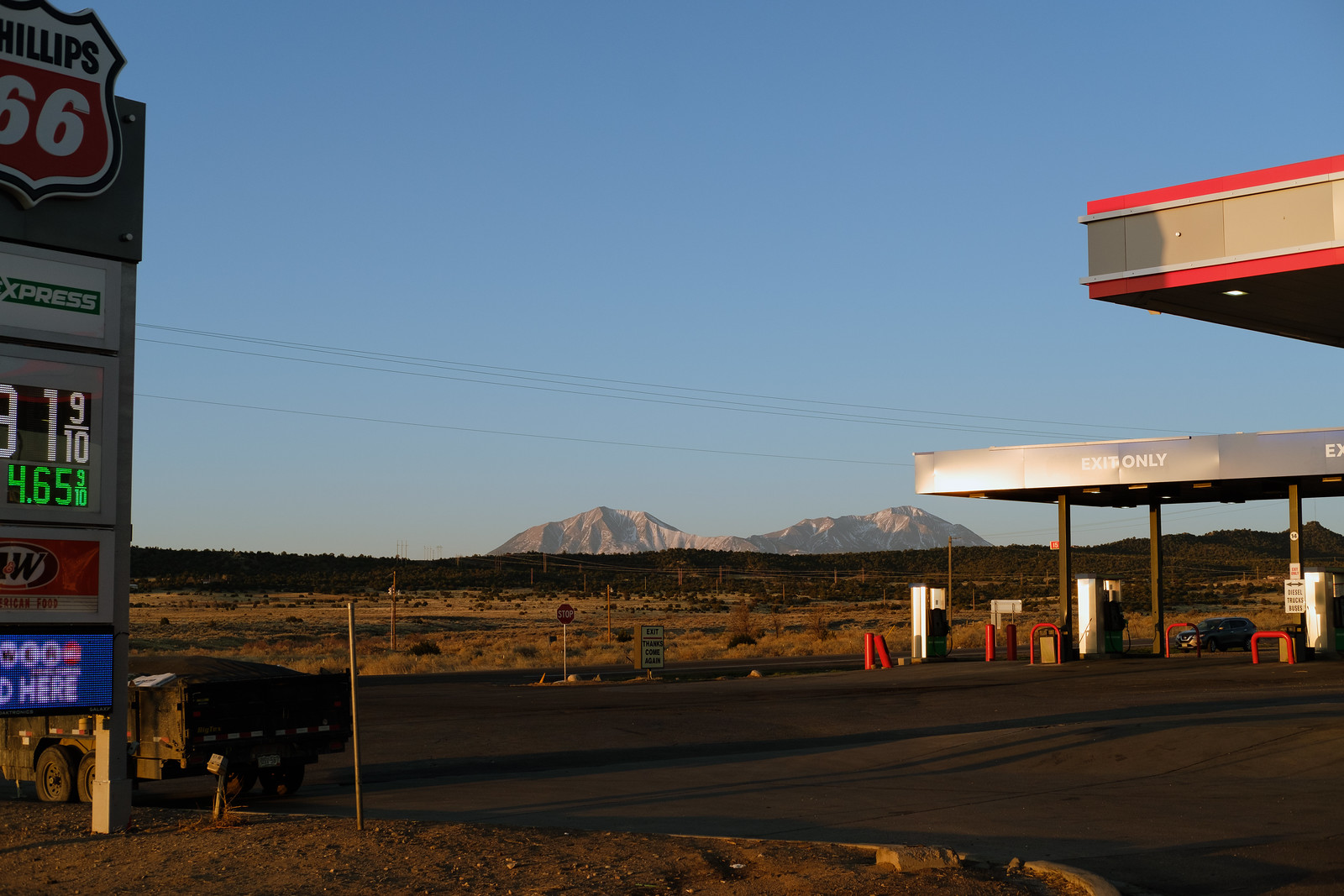This photograph captures a clear blue desert landscape dominated by a gas station. The sky is an uninterrupted expanse of blue, with no clouds visible. In the middle distance, a series of mountaintops rise prominently, flanked by power lines. The foreground features an empty gas station with three visible gas pumps under a canopy. The station is identified by a Phillips 66 sign displaying the word "Express" and a gas price of $4.65. A vehicle is parked near a display of advertisements on the left side of the image. Surrounding the gas station are flat, grassy areas and a scattering of trees, adding a touch of greenery to the sandy desert backdrop. Further in the distance, an SUV is seen driving along the roadway leading up to the gas station.